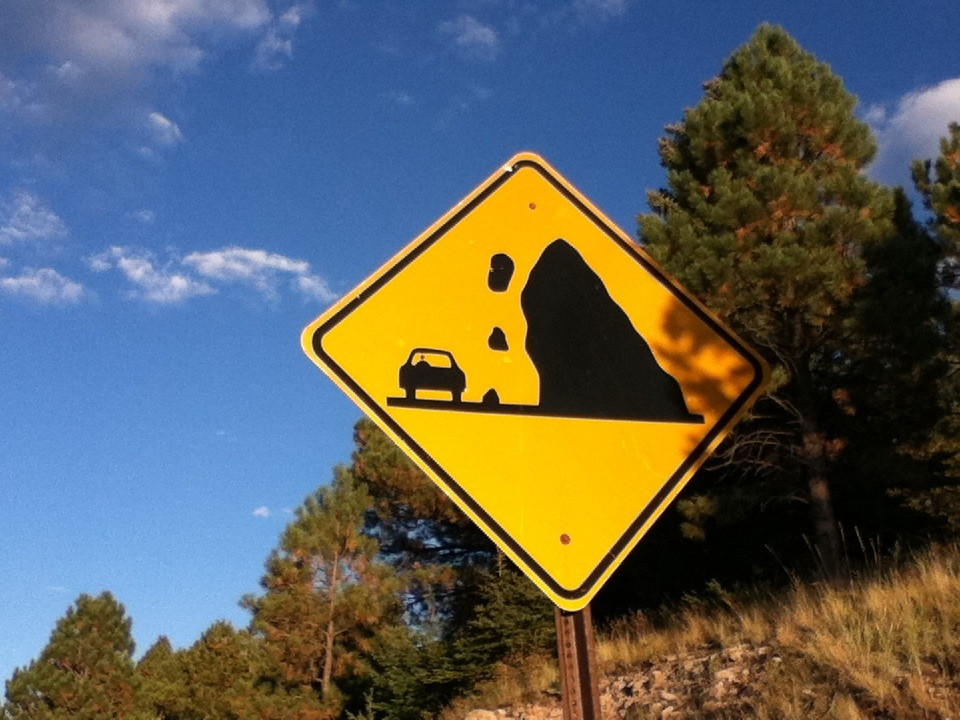This photograph captures a vividly detailed outdoor scene featuring a warning sign indicating the potential for rock slides. The vibrant yellow, diamond-shaped sign is mounted on a rusty, brown post that rises from the bottom of the frame. The sign's black illustration depicts a car beside a steep cliff with three large boulders tumbling down, suggesting the danger of falling rocks in the area. The background showcases a picturesque setting with a deep blue sky speckled with a few fluffy white clouds. Surrounding the sign, there is a tree line dominated by tall, green pine trees that ascend a rocky hill, interspersed with some brownish rocks and patches of green and brown grass. The entire composition situates the viewer firmly in a natural, scenic, yet potentially hazardous environment.